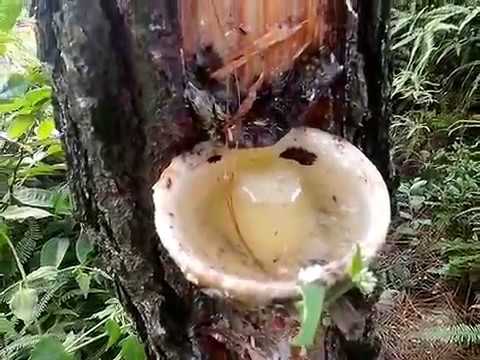The photograph depicts an outdoor scene featuring a pine tree from which resin is being extracted. At the center of the image, a white bowl-shaped container, possibly made of porcelain, has been affixed to the tree trunk to collect the resin. The bowl, glossy and somewhat resembling an inverted suction cup or a natural mushroom, appears slightly dirty and contains a glue-like white liquid, indicative of the pine resin. The pine tree's trunk is partially stripped of its bark, exposing its dark, almost blackened surface, which emphasizes the extraction site. Surrounding the trunk is a mix of green vegetation, including ferns and petal-like leaves, with scattered yellow and brown foliage, confirming the natural outdoor setting.